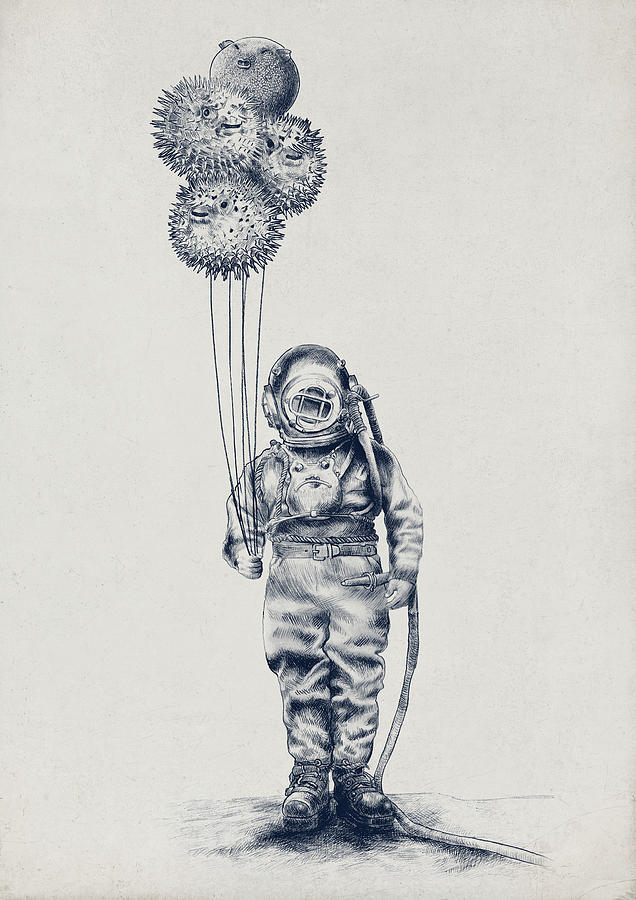This is a detailed, black-and-white pencil illustration depicting a man in early 1900s-style scuba gear, characterized by a heavy metal helmet with cross-hatched glass plates on the face. The diver, wearing bulky boots and traditional diving suit, is standing on a subtly shaded, sandy ocean floor. His right hand holds four puffer fish on strings, floating like balloons, with one of the top fish resembling a blown-up pig. The background is predominantly white, emphasizing the central figure and the surreal quality of the scene.